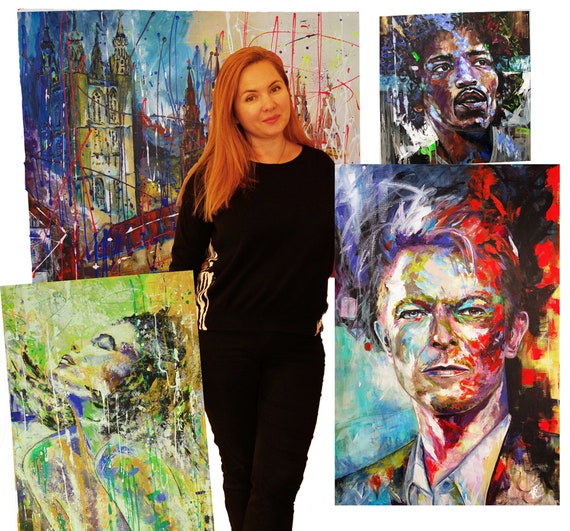In this captivating collage, a striking woman with long, side-parted red hair stands centrally, dressed in a sleek all-black long-sleeve dress. She is surrounded by four expressive paintings with a distinct splash-art style, reflecting vibrant, splattered colors. Behind her, a large canvas mural depicts a cityscape with various buildings in an abstract storm of colors. In the upper right corner, a smaller square painting showcases Jimi Hendrix's head, adorned with lively blues and browns in a splattered style. Below this, in the lower-right corner, David Bowie's torso portrait stands out in a horizontal rectangle, featuring multicolored splashes with contrasting hues of red, black, teal, and white. On the lower left, another horizontal rectangle painting portrays a woman with dark hair, eyes closed, captured in green and yellow tones, with a serene, upward gaze. This artistic scene blends music and visual art, offering a dynamic and vibrant homage to iconic figures.